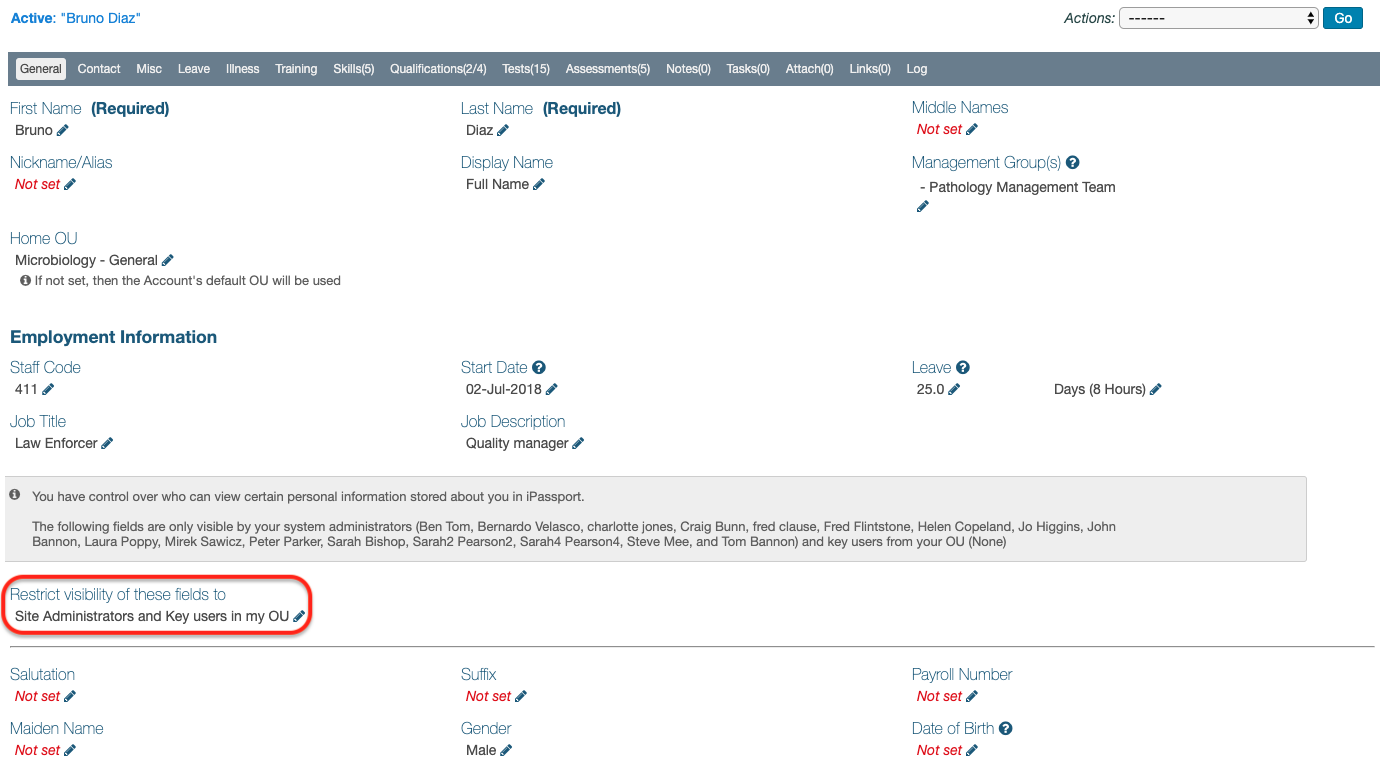**Detailed Caption of Screenshot:**

The screenshot depicts a section of a webpage, primarily focused on a user profile or account settings interface. 

### Header:
- At the top left, there's a blue text segment stating **"Active Bruno Diaz"** in quotation marks.
- On the top right, it says **"Actions"** with a drop-down menu symbolized by six hyphens.
- Adjacent to the drop-down menu, there's a blue button labeled **"Go"** in white text.

### Navigation Banner:
- Below the header, there’s a blue-gray navigation banner with multiple selectable options:
  - **General** (selected, highlighted with a gray box)
  - **Contact**
  - **Misc**
  - **Leave**
  - **Illness**
  - **Training** (with 5 in parentheses)
  - **Skills** (with 5 in parentheses)
  - **Qualifications** (2 out of 4 in parentheses)
  - **Tests** (15 in parentheses)
  - **Assessments** (5 in parentheses)
  - **Notes** (0 in parentheses)
  - **Tasks** (0 in parentheses)
  - **Attached** (0 in parentheses)
  - **Links** (0 in parentheses)
  - **Log**

### User Details:
- There are multiple rows containing the user's information, structured in labeled text fields:
  - **First Name**: In blue text followed by **"Required"** in bold, displaying **"Bruno"**.
  - **Last Name**: In blue text followed by **"Required"** in bold, displaying **"Diaz"**.
  - **Middle Name(s)**: In blue text followed by **"Not Set"** in red text.
  - **Nickname / Alias**: In blue text followed by **"Not Set"** in red text.
  - **Display Name**: **"Full Name"**
  - **Management Group**: In parentheses, **"Pathology Management Team"**
- Another row includes more professional information:
  - **Home OU**: **"Microbiology - General"** with an informative note stating *"If not set, then the account's default OU will be used."*
  - **Employment Information**:
    - **Staff Code**: **"411"**
    - **Start Date**: **"02 July 2018"**
    - **Leave**: **"25.0 days (8 hours)"**
    - **Job Title**: **"Law Enforcer"**
    - **Job Description**: **"Quality Manager"**

### Security and Visibility Settings:
- There's a gray box indicating **"You have control over who can view personal information about you."**
- It lists system administrators and key users who can see the information:
  - **Ben Tom**
  - **Bernardo Velasco**
  - **Charlotte Jones**
  - **Craig Bunn**
  - **Fred Claus**
  - **Fred Flintstone**
  - **Helen Copeland**
  - **Joe Higgins**
  - **John Bannon**
  - **Laura Poppy**
  - **Amiric Savicks**
  - **Peter Parker**
  - **Sarah Bishop**
  - **Sarah 2 Pearson**
  - **Sarah 4 Pearson**
  - **Steve Me**
  - **Tom Bannon**
  - and key users from the user's OU (None specified)
- A red box demarcates this section with the label **"Restrict visibility of these fields to"**, followed by **"Site Administrators and Key Users in my OU."**
  
### Additional Information:
- **Salutation**: **"Not Set"**
- **Suffix**: **"Not Set"**
- **Payroll Number**: **"Not Set"**
- **Maiden Name**: **"Not Set"**
- **Gender**: **"Male"**
- **Date of Birth**: **"Not Set"**

This detailed description provides an exhaustive breakdown of the interface elements and user-specific information contained within the screenshot.